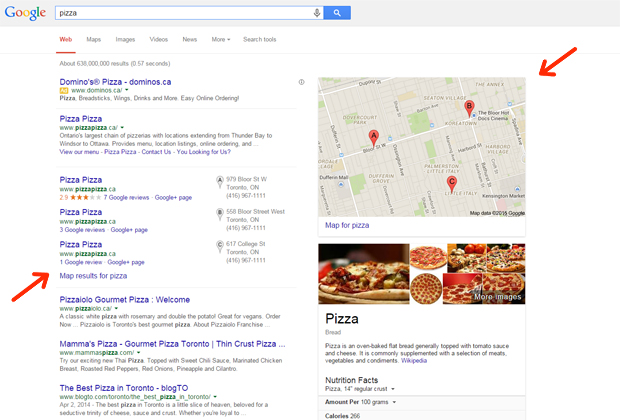This image depicts a Google search results page for the query "pizza." At the top, the search bar clearly displays the word "pizza," and the "web" tab is highlighted in red and underlined. The first search result is a paid advertisement for Domino's Pizza, noticeable by the accompanying "Ad" icon. Following this is a series of organic search results, starting with several listings for "Pizza Pizza." A red arrow has been drawn to emphasize one of these "Pizza Pizza" results, directing attention to it. 

Further down, the search results include listings for "Pizza Lolo Gourmet Pizza," "Mama's Pizza," and a guide on "the best pizza in Toronto." To the right of these results, there is a Google map showing locations labeled A, B, and C, corresponding to the search results. Below the map, there are thumbnail images showcasing different types of pizza. Towards the bottom right of the page, a succinct definition of pizza is provided, sourced from Wikipedia: "Pizza is an oven-baked flatbread generally topped with tomato sauce and cheese, commonly supplemented with a selection of meats, vegetables, and condiments."